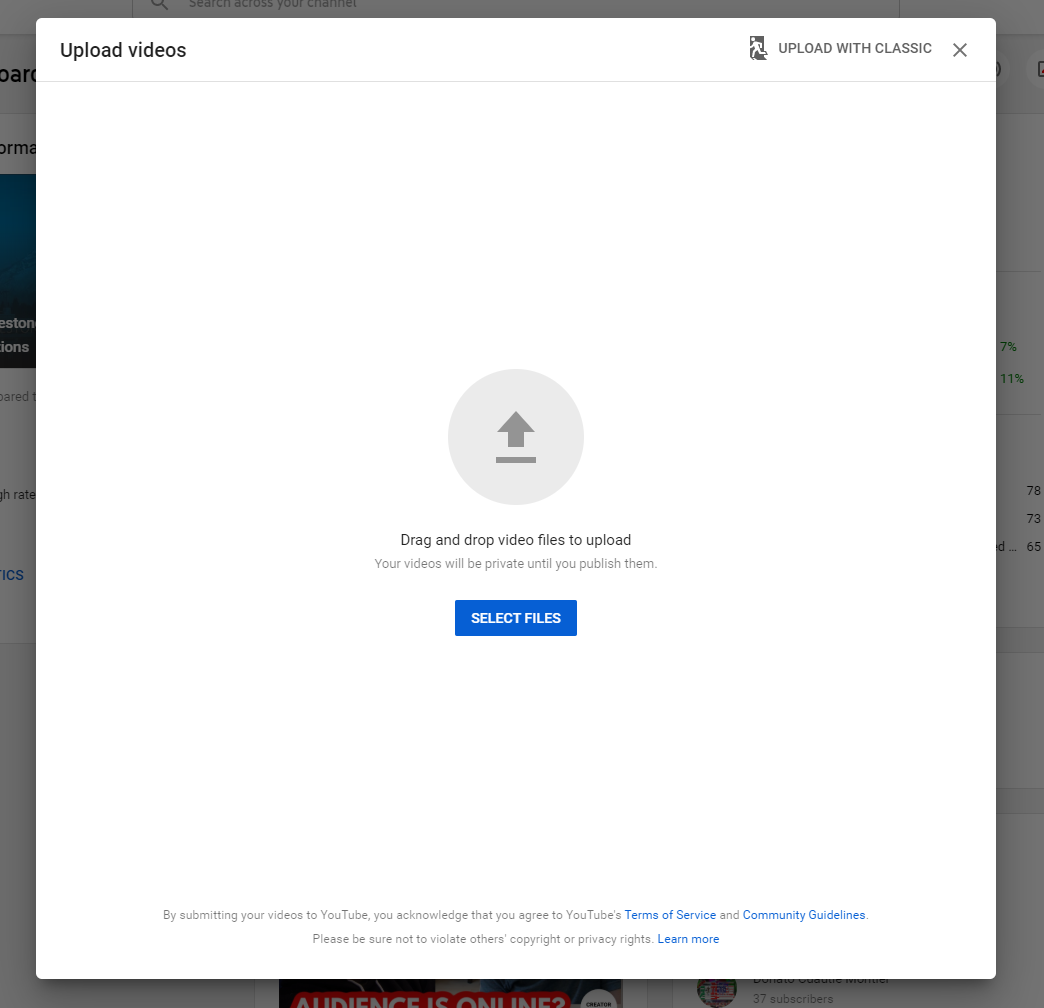In this image, we see a pop-up window for video uploads positioned on the upper left corner of the screen. At the top right of this window, there’s a text indicating "UPLOAD WITH CLASSIC" in all capital letters and gray font, accompanied by a close "X" symbol. Adjacent to this, on the left, is a silhouette icon of a man running leftward against a gray background. 

Central to the pop-up is a prominent gray circle with a darker gray arrow pointing upward, symbolizing the upload action. Directly beneath this arrow is a horizontal gray line, coupled with the instruction "Drag and drop video files to upload" below. Lastly, at the bottom of the window, there is a blue button labeled "Select Files," where users can click to upload their videos.